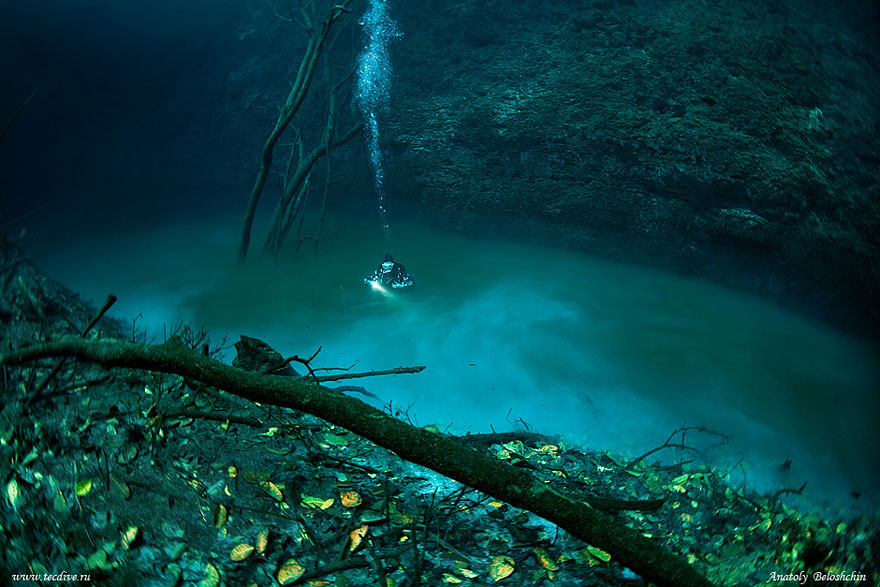The image depicts a scuba diver submerged underwater, equipped with a black diving suit. Bubbles ascend from the diver’s head, indicating active breathing. The scene has a blue-greenish hue and appears to be dimly lit, suggesting an underwater environment, possibly a riverbed. A long, slender tree trunk or branch extends across the foreground, and scattered green leaves are visible on the riverbed floor. The surroundings feature rock formations, adding to the rugged terrain. Moss-like vegetation can be seen along the back wall of the underwater scene. A notable feature in the bottom of the image are fragments of tree limbs and vegetation, further supported by a watermark "www.techdive.ru" which confirms the underwater context. Overall, the image captures a murky, submerged world with the diver exploring a potentially seasonal or flooded area characterized by underwater trees and natural debris.